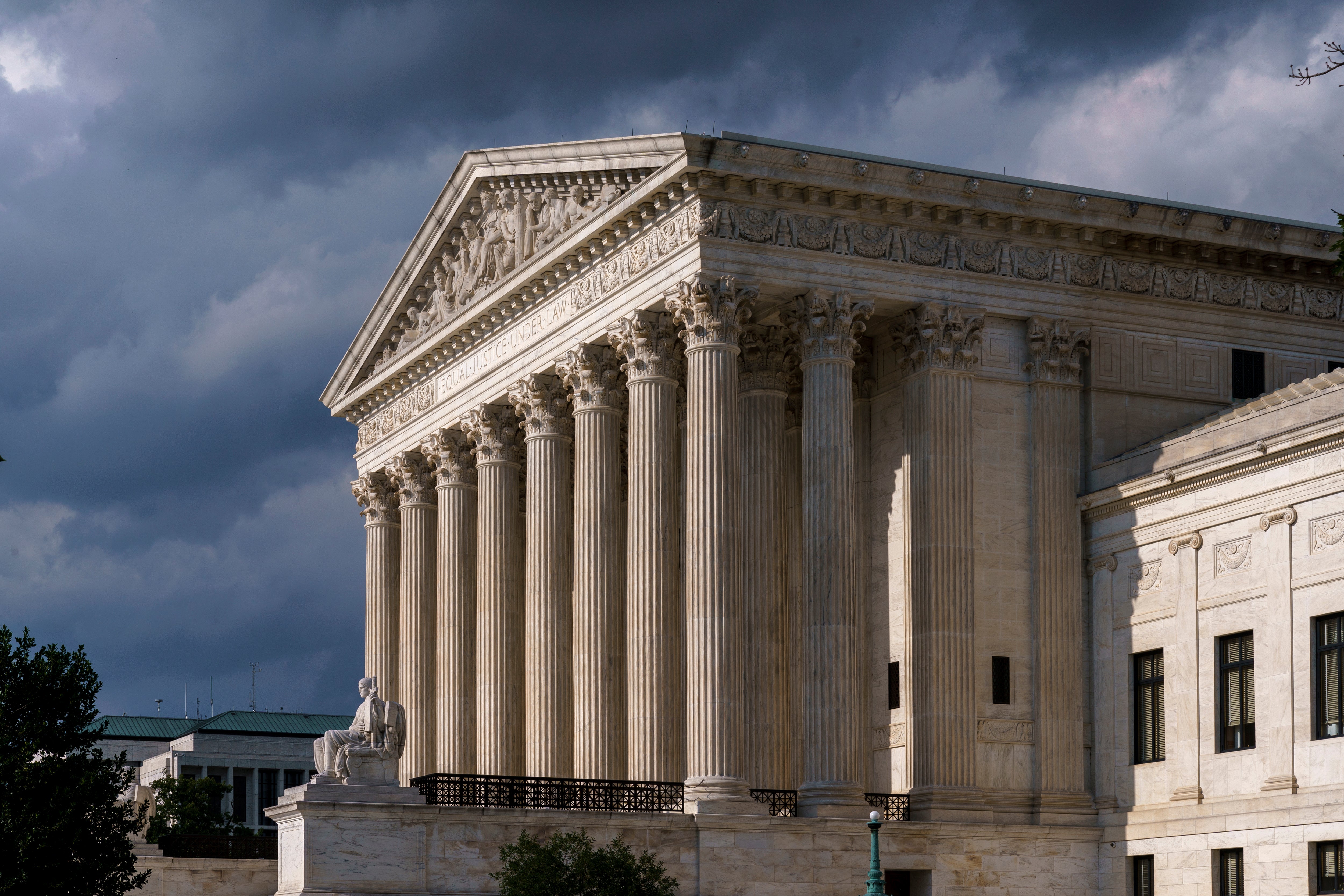The image depicts an imposing building in classical Roman or Greek architectural style, reminiscent of courthouses or government buildings like the US Supreme Court or the Capitol building. The structure features a prominent façade with at least ten Roman-style columns with vertical grooves. These columns support a dramatically sloped triangular roof adorned with ornate decorations, possibly depicting scroll designs or historical scenes. Inscribed along the top is a phrase related to justice, suggesting that this is indeed a courthouse. A lifelike statue of a seated human figure is positioned in front of the building, adding to the gravitas of the scene.

The building extends sideways, revealing additional sections with numerous vertically aligned rectangular windows framed in black. The construction material appears to be either white bricks or white marble, giving it a pristine and authoritative appearance. Surrounding the building are patches of greenery, including bushes and tree branches, providing a contrast to the light brown stone wall at the lower level.

Above, the sky is ominous, filled with large, menacing clouds of dark gray and hints of lighter gray and white, indicating an impending storm. The overall atmosphere suggests a typically solemn and formal setting, underscored by the stormy weather.